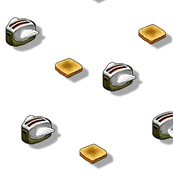This image is a whimsical illustration that depicts a repeated pattern of small, silver toasters with short, white angel wings adjacent to slices of toast. The background is completely white, creating the illusion that both the toasters and toast are floating. Each toaster has a front silver panel and a gray bottom section. A slight orange tint around the toaster slots suggests they might be on. Shadows under each toaster and slice of toast enhance the floating effect. The toast is lightly browned in the center with white edges, and each piece of bread displays varying degrees of toasting, with some areas slightly burnt. The arrangement follows a diagonal pattern across the image, sometimes irregular in spacing, featuring a total of four toasters and three slices of toast. The overall aesthetic resembles a quirky, animated wallpaper design.